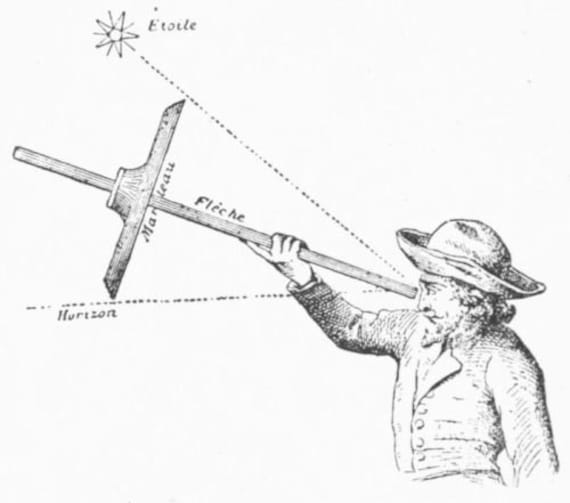A detailed pen and ink illustration, likely dating from the 18th or early 19th century, presents a side profile view of a man using a wooden gauging device. The man, who has curly shoulder-length hair, a full beard, and wears an old-fashioned hat along with a buttoned coat and bowtie, holds the device with his right hand up to his eye. The wooden apparatus, similar in length to a yardstick but thicker, features a wider piece crossing over the top, resembling a drafting T-square. From the man's eye, lines extend outward, labeled "Étoile" (star) at the top, "Fleche" (arrow) in the middle, and "Horizon" at the bottom, suggesting the device is used to measure spatial placement. The illustration, which may have been reproduced as a photograph, also includes an eight-pointed star symbolizing the sun, hinting at its possible use as an early timing or navigation tool. The meticulous detailing and schematic style evoke the technical illustrations of past centuries.